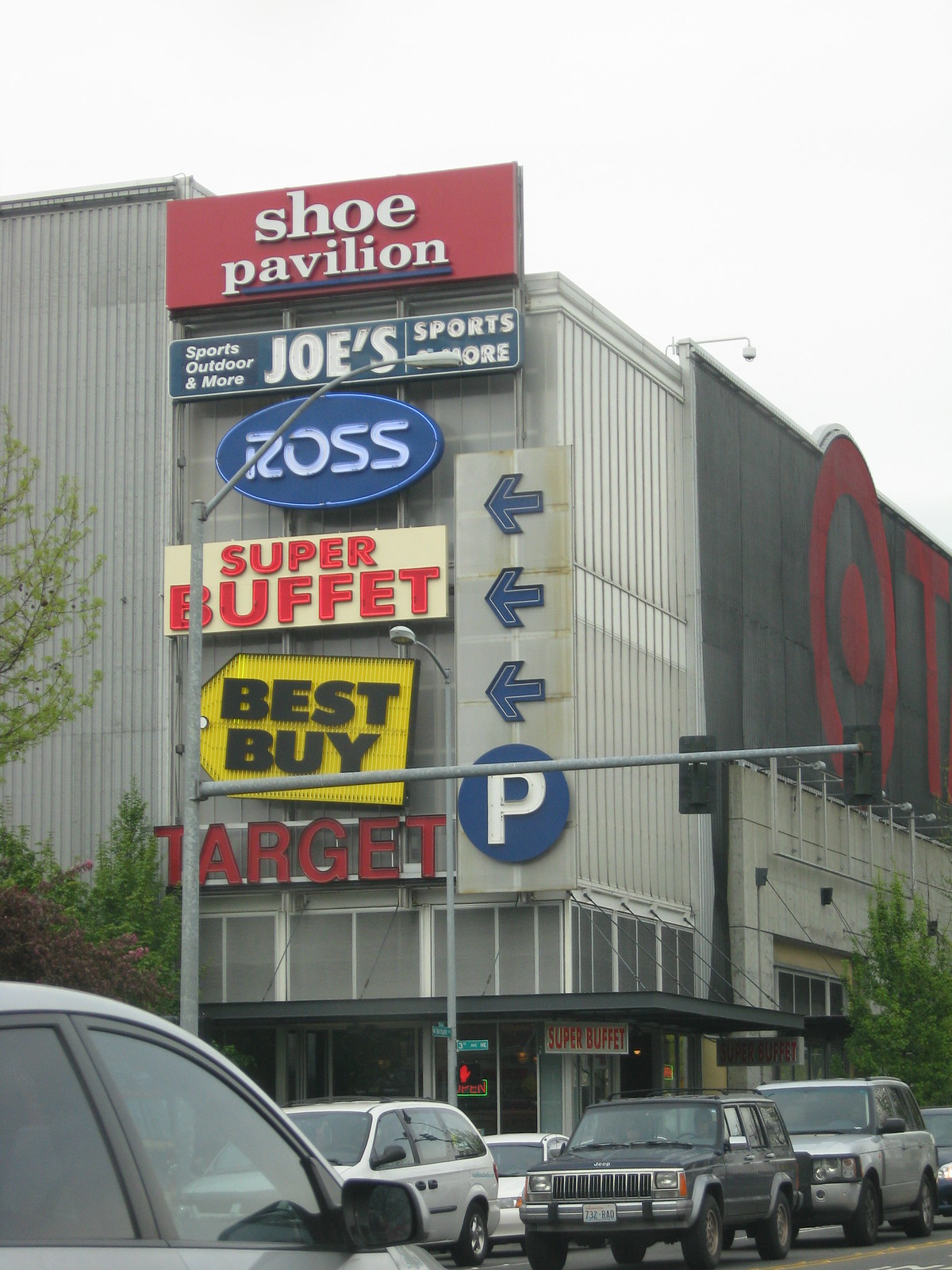A bustling city street scene captures a busy thoroughfare lined with various stores and abundant pedestrian activity. At the forefront stands a multi-story building showcasing a multitude of retail signs arranged from top to bottom: "Shoe Pavilion," "Sports Outdoor and More," "Joe's Sports and More," "Ross," "Super Buffet," "Best Buy," and at the bottom "Target," recognizable by the distinctive bullseye logo and red "T" on the building's facade.

Across a busy street teeming with cars in motion, a prominent streetlight and a large circular parking sign with directional arrows point the way to the designated parking area. The structure itself is a muted gray, contrasted by pockets of greenery with trees visible on the left.

This vibrant photograph encapsulates the dynamic atmosphere of an urban shopping center, highlighting not only the well-known retail establishments but also the hustle and bustle of city life.